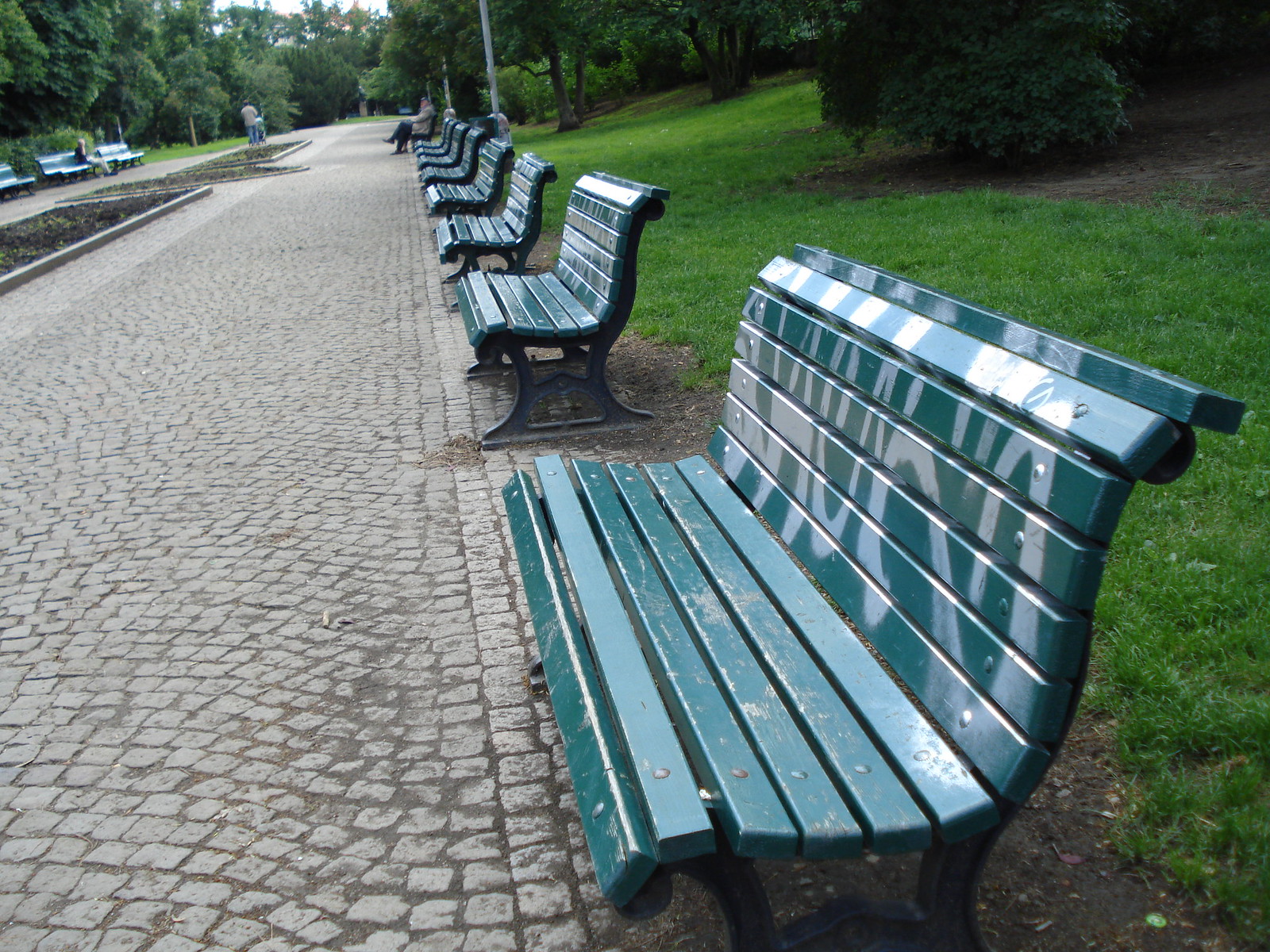The image captures a serene scene along a wide walkway in a public park, framed by cobblestones arranged in a semi-circular design that stretches from the bottom left to the center top of the photo. The main focus is a row of forest-green wooden benches, which stand diagonally from the bottom right to the background. The closest bench, positioned at the bottom center, shows signs of white spray-painted graffiti, a pattern repeated on some of the other benches, indicating wear and vandalism.

To the right of the benches is a lush grassy incline with dark green bushes at the top, adding a natural backdrop. Distant streetlight bases and trees provide depth, while a faint silhouette of a man in a brown jacket and black pants is visible at the far end of the row, seated on a bench. The left side of the walkway features more benches facing each other, with one bench in the top left corner occupied by another person. The setting is bathed in daylight, with planters seen alongside the cobblestone path, suggesting a well-maintained area ideal for relaxation and solitude.